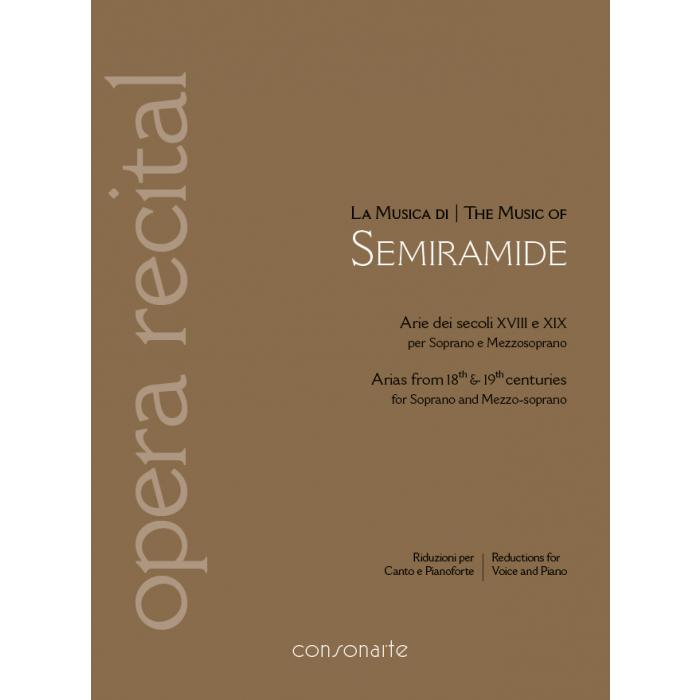The image displays the cover of a booklet or pamphlet with a light brown background. On the left side, oriented from bottom to top, large white letters spell out "Opera Recital." Along the right side, in the center, black letters read "La Musica di" followed by "The Music of Semiramide" in large white letters. Below this, black text states "Erie de Sicoli XVIII XIX per soprano e mezzo-soprano," which translates to "Arias from the 18th and 19th centuries for soprano and mezzo-soprano." Near the bottom right, it reads "Riduzioni per canto e pianoforte," translated as "Reductions for voice and piano." At the very bottom, centered in white letters, is the word "Consonante."